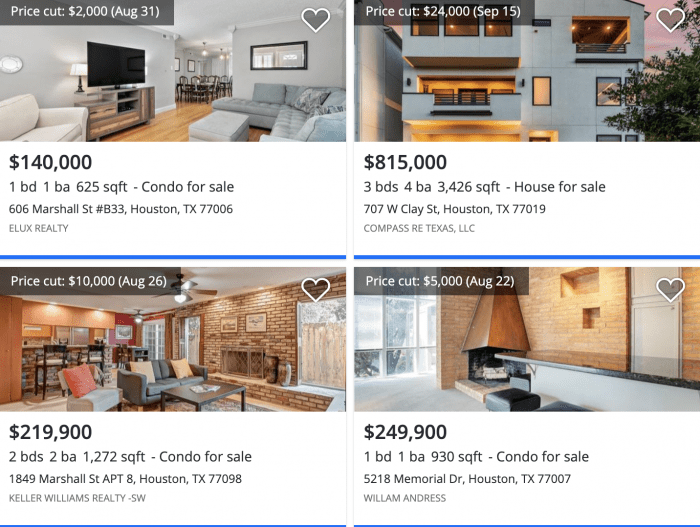For sale: A charming 1-bedroom, 1-bathroom condo located at 606 Marshall Street, Unit B33, Houston, TX 7701. Priced at $140,000, this 675 square foot unit offers a cozy living space perfect for singles or couples. Featuring modern amenities, the condo is situated in a desirable neighborhood with convenient access to local attractions and services. Don't miss out on the opportunity to own this inviting property in the heart of Houston.